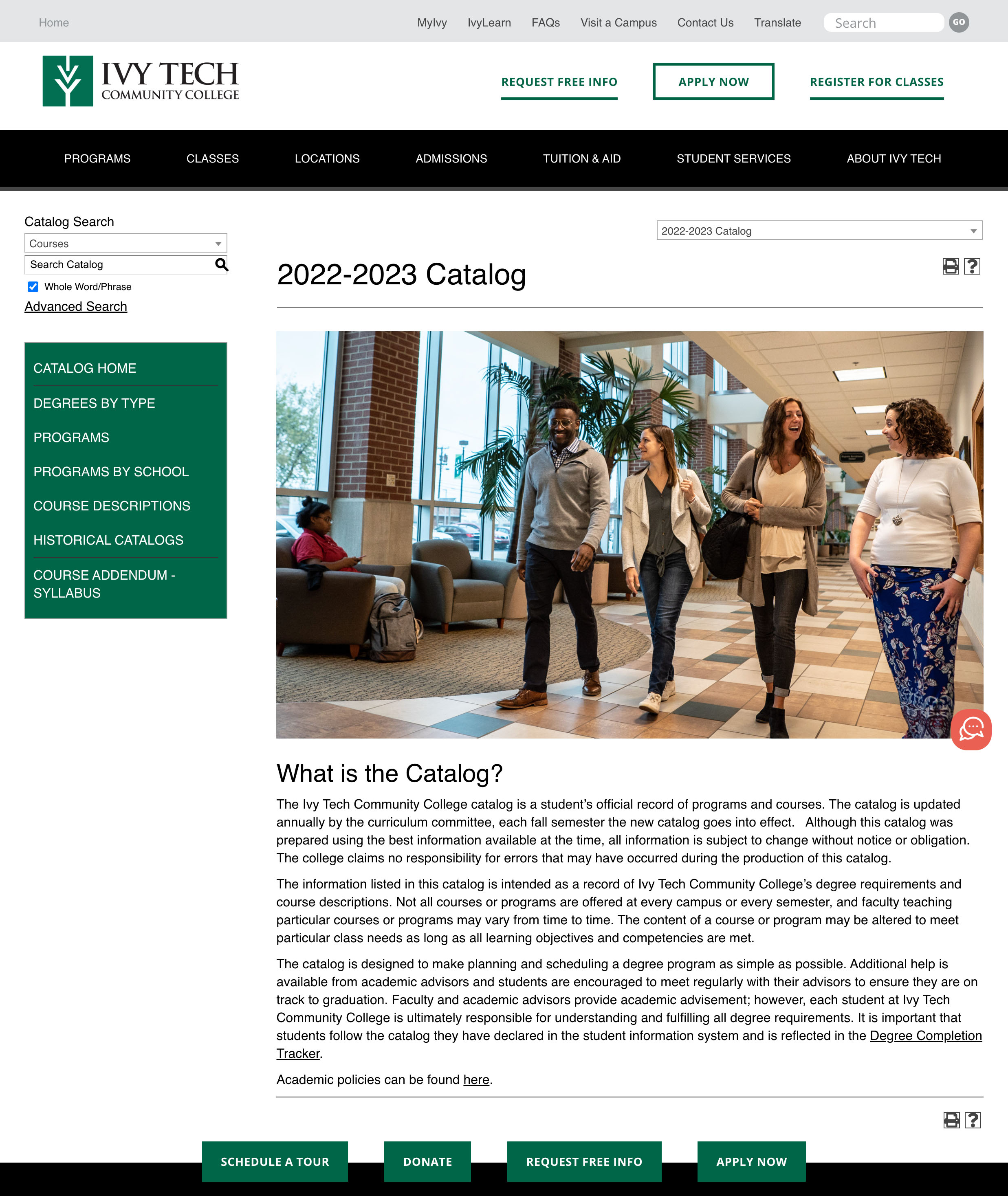The image prominently features the Ivy Tech Community College website interface. In the top left corner, there is a green and white logo that reads "Ivy Tech Community College." Adjacent to the logo, the header menu includes the following options: "MiLearn," "FAQs," "Visit Campus," and "Contact Us." A search box is placed nearby, followed by a button labeled "Request Free Info." Additionally, there is an "Apply Now" button and a link titled "Register for Classes."

Beneath this section, a black navigation bar contains links to various important sections: "Programs," "Classes," "Locations," "Admissions," "Tuition and Aid," "Student Services," and "About Ivy Tech." Further down, the screen displays the title "2022-2023 Catalog." Below this, a photograph captures three women and one man strolling down a hallway. Accompanying the image, text reads, "What is the Catalog? The Ivy Tech Community College Catalog is a student’s official record of programs and courses. The Catalog is updated annually by the Curriculum Committee," although the remaining text appears too blurry to decipher.